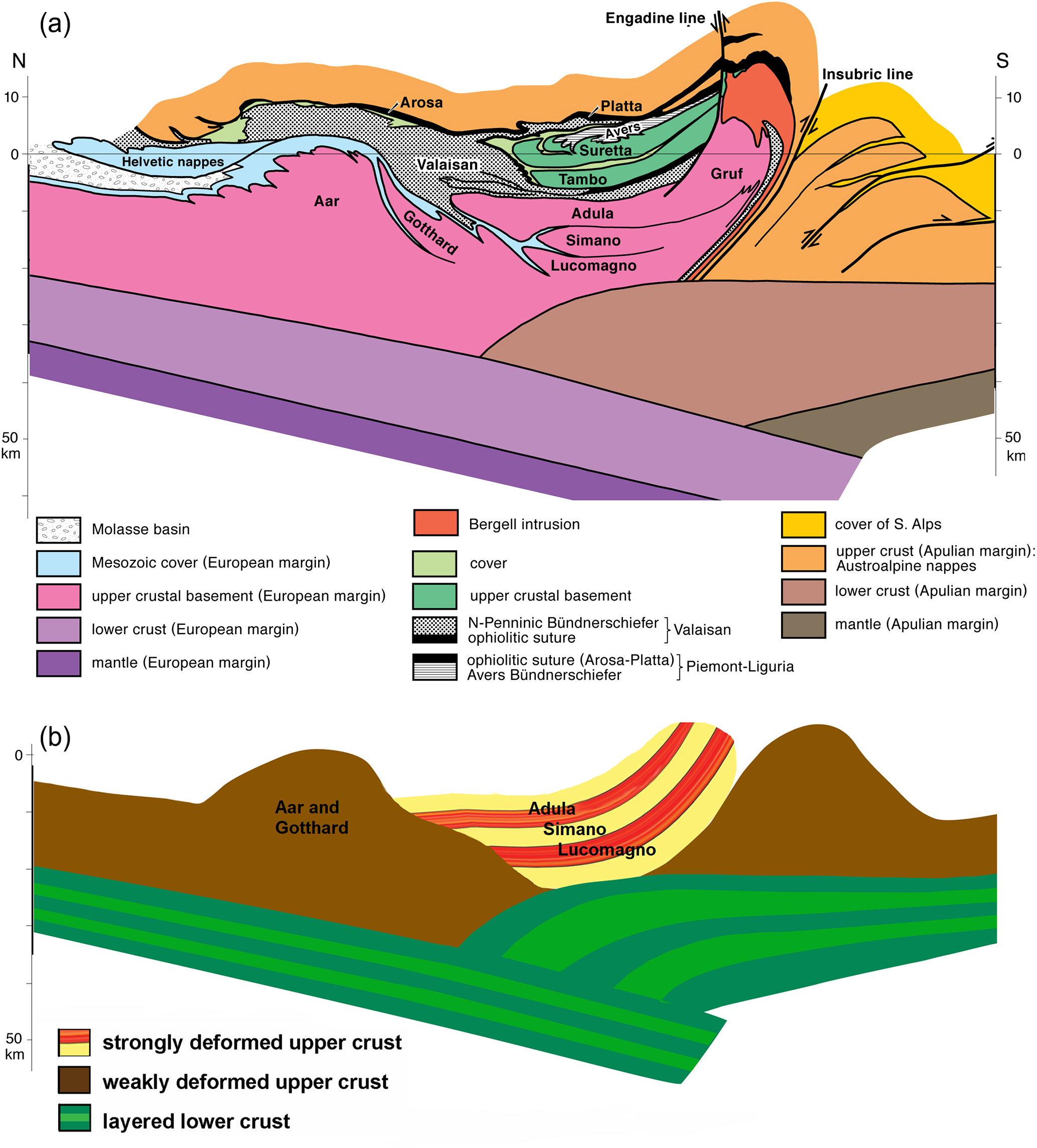The image is a detailed diagram of different layers of the Earth's crust, split into two sections labeled A and B. Section A, occupying the top half, features a complex arrangement of colors with corresponding labels and explanations. It includes multiple vertical lines marked with reference points—both labeled X with "N" and "S" at the respective tops—and kilometric breakdowns. The colors represented include pink, purple, light purple, brown, beige, orange, yellow, mustard, blue, turquoise, white, gray, and involve locations or geological entities such as Hivetic Neibs, Arosa, Plata, Engadin line, Innsbruck line, Graf, Adula, Simano, Lukomagno, Gotthard, Tambo, Sureta, Balaisan. Each color signifies different geological features described at the graph's bottom. Examples include Molasse Basin, Mesozoic Cover European Margin, Upper Crustal Basement European Margin, Lower Crust European Margin, Mantle European Margin, Burgle Intrusion, Cover, and Ophiolite Suture among others.

Section B, smaller and located beneath section A, features a simpler construction with a single vertical line on the left. It includes three distinct color bands: a yellow and red combination, brown, and a light and dark green combination. This section labels geological features known as Ar, Gotthard, Adula, Simano, and Lukomagno, with the color codes indicating Strongly Deformed Upper Crust, Weakly Deformed Upper Crust, and Layered Lower Crust. 

Overall, the diagram serves as an intricate representation of Earth's crust layers, with a detailed key explaining the significance of each color and feature.